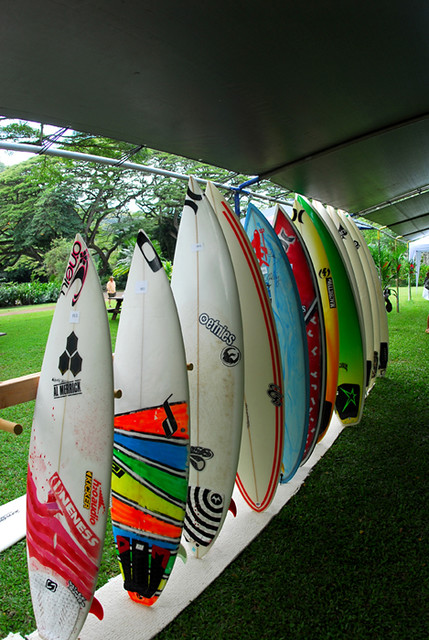This outdoor photograph showcases an impressive display of about a dozen surfboards standing upright, organized in a simple wooden rack under a dark gray canopy. Positioned on a well-trimmed green lawn, the surfboards are neatly lined up from left to right, with shorter boards in the front and longer ones at the back. Each surfboard is unique, featuring a variety of colors and designs, though many share a white base. The frontmost surfboard is off-white with a red liquid design, followed by a white board with vibrant orange, blue, green, and yellow stripes. Behind them stands a largely white board adorned with black circles and another with red striping details. The collection also includes solid red, green, and blue surfboards, among others with colorful patterns. The display appears to be part of a stall or demonstration, possibly related to a surf contest, as suggested by the temporary pop-up structure. In the background, well-maintained shrubs, lush leafy trees, and a brown park bench provide a serene, park-like setting. The surfboards are both aesthetically pleasing and seemingly well-kept, adding to the organized and vibrant outdoor scene.